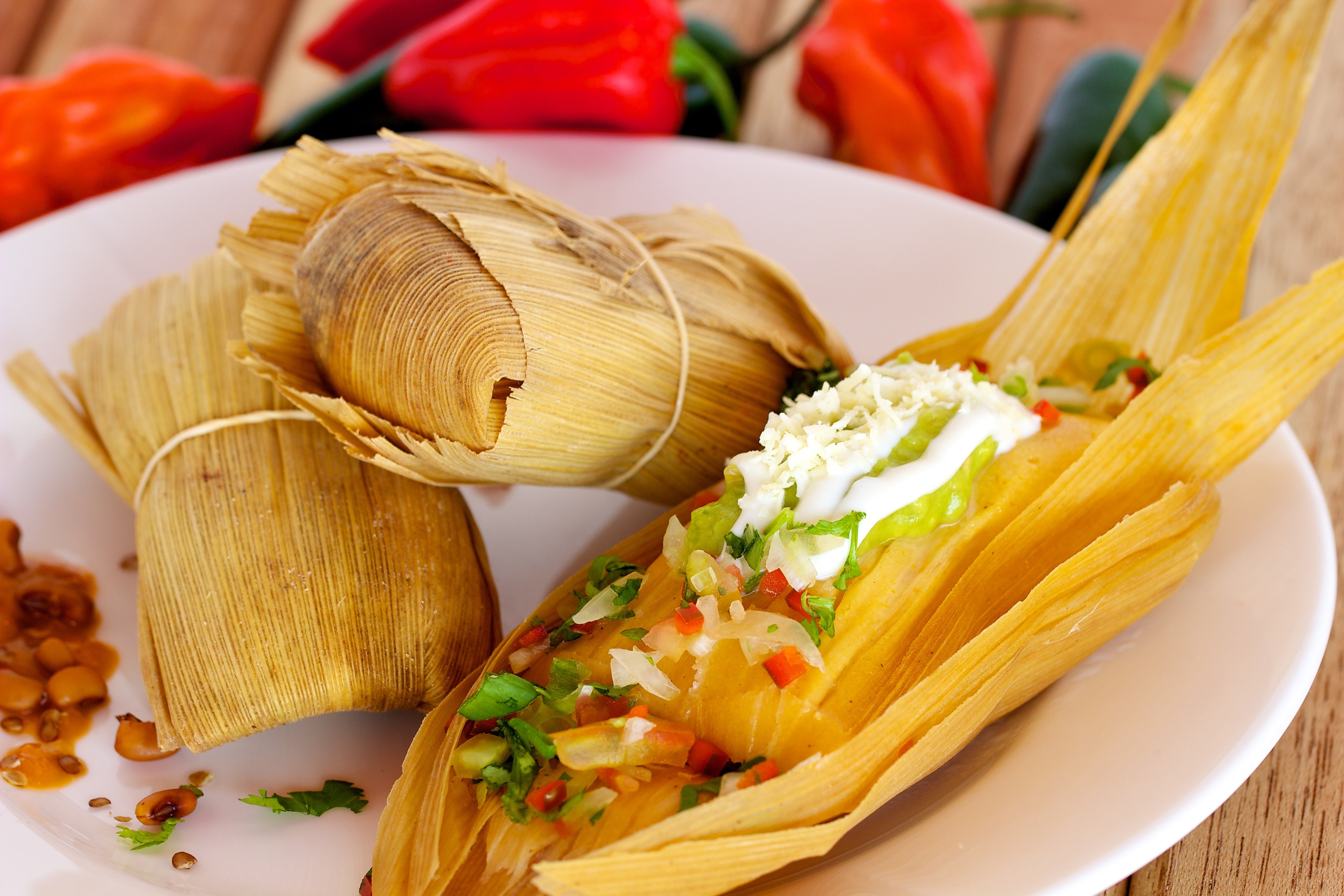This is a color photograph of a tastefully staged close-up of three tamales meticulously arranged on a large, white ceramic plate. Two tamales remain wrapped in their outer corn husks, neatly secured with rubber bands, while the third tamale lies open, revealing a vibrant mix of fillings. The open tamale showcases a colorful combination of salsa fresca, fresh cream, guacamole, and sprinkled cheese, displaying a palette of green, red, and white. Accompanying the tamales, a sparse serving of beans is placed in the left-hand corner of the plate, contributing to the presentation. Red chilies and peppers subtly frame the plate, with a red pepper prominently positioned with a green stem, enhancing the aesthetic appeal. The background appears blurred, ensuring the focus remains on the tamales. This professionally taken photograph captures a modern and appetizing presentation of the dish, emphasizing its fresh ingredients and careful arrangement.